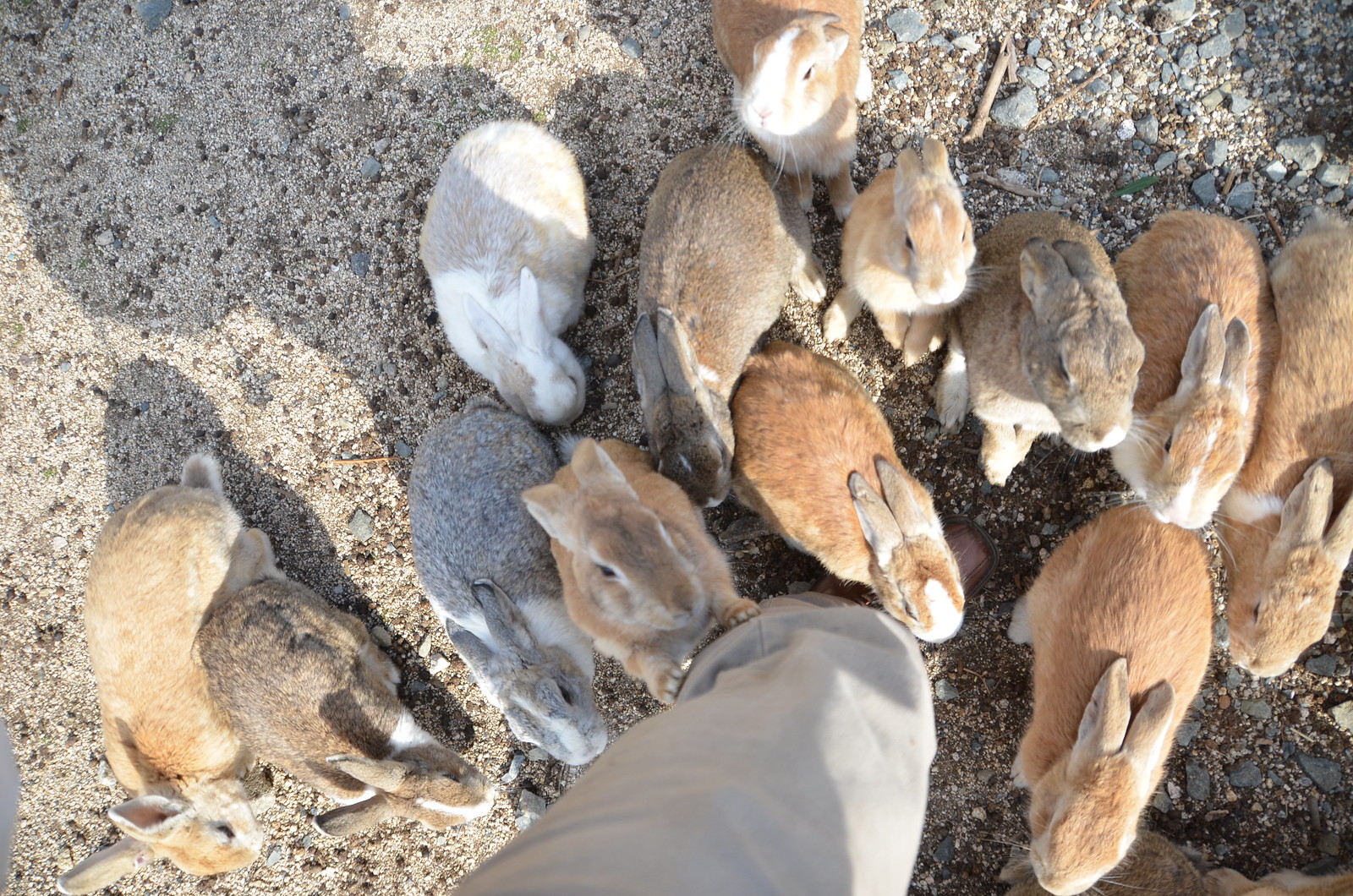In this photograph, we see a group of approximately 12 to 13 small rabbits, mainly Netherland Dwarf-like rabbits, huddled together around the leg of a human. The human is wearing light grayish khaki pants and brown shoes, casting a shadow on the sandy, pebble-strewn ground beneath them. The rabbits exhibit various colors, with the majority being a light brown hue with white highlights. Among them, there is a distinct gray rabbit and another that is almost entirely white with some light tan markings. One rabbit stands out by standing up against the human's leg. The setting appears to be outdoors, and the rabbits' dense clustering around the leg suggests a sense of curiosity or comfort. The human's leg serves as a central focal point around which the diverse and furry group of rabbits is gathered, highlighting their unique colors and playful behavior.